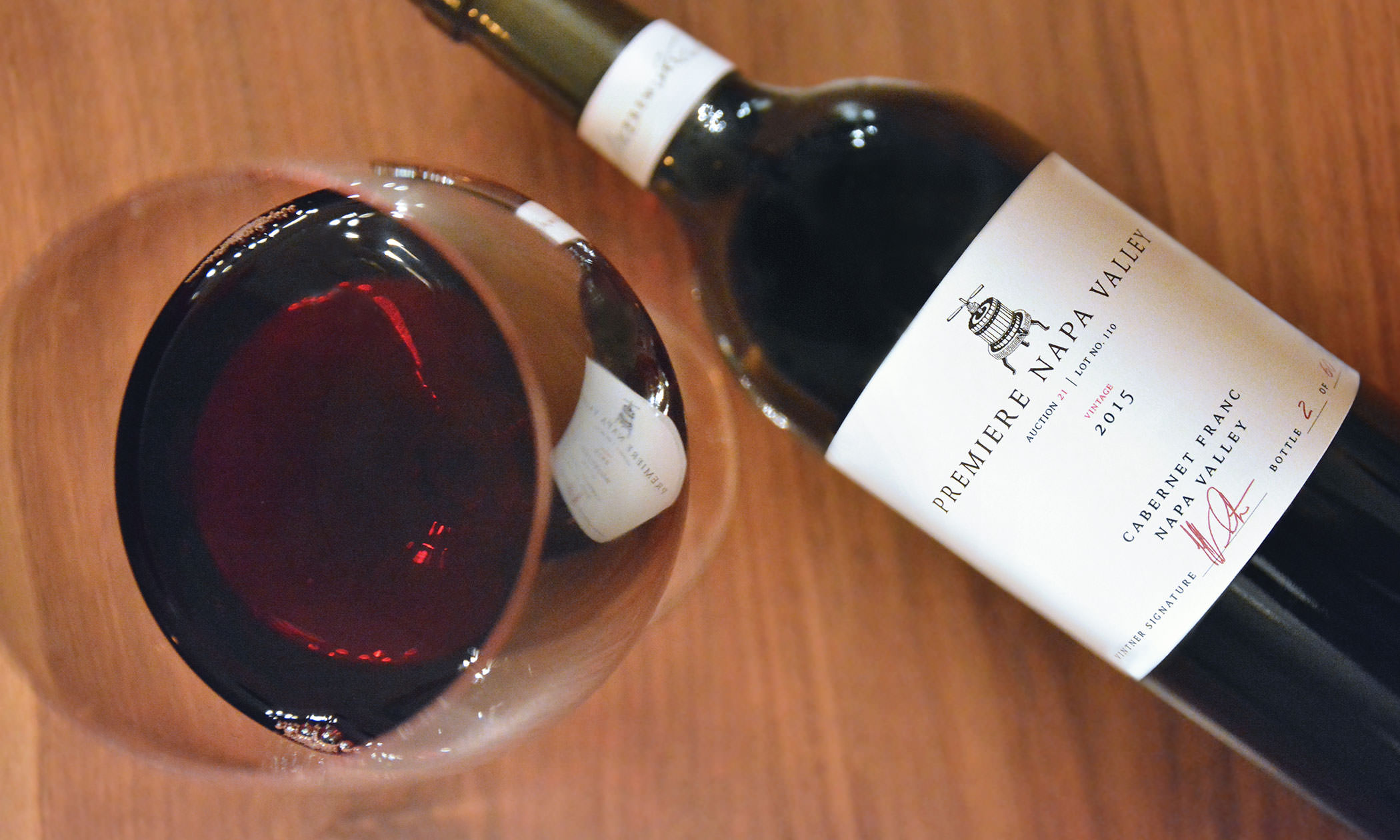This aerial close-up image showcases a bottle of Premier Napa Valley Cabernet Franc 2015 wine laying flat on its side on a wooden table, with its detailed white label featuring the name and a picture of a wine barrel clearly facing the camera. The label is prominently displayed, though only part of the bottle is visible while the top and bottom are out of frame. Positioned to the left of the bottle is a half-full stemmed wine glass containing dark red wine with visible bubbles, casting a reflection of the bottle on its side. The entire scene is captured from above, emphasizing the rustic elegance of the presentation.